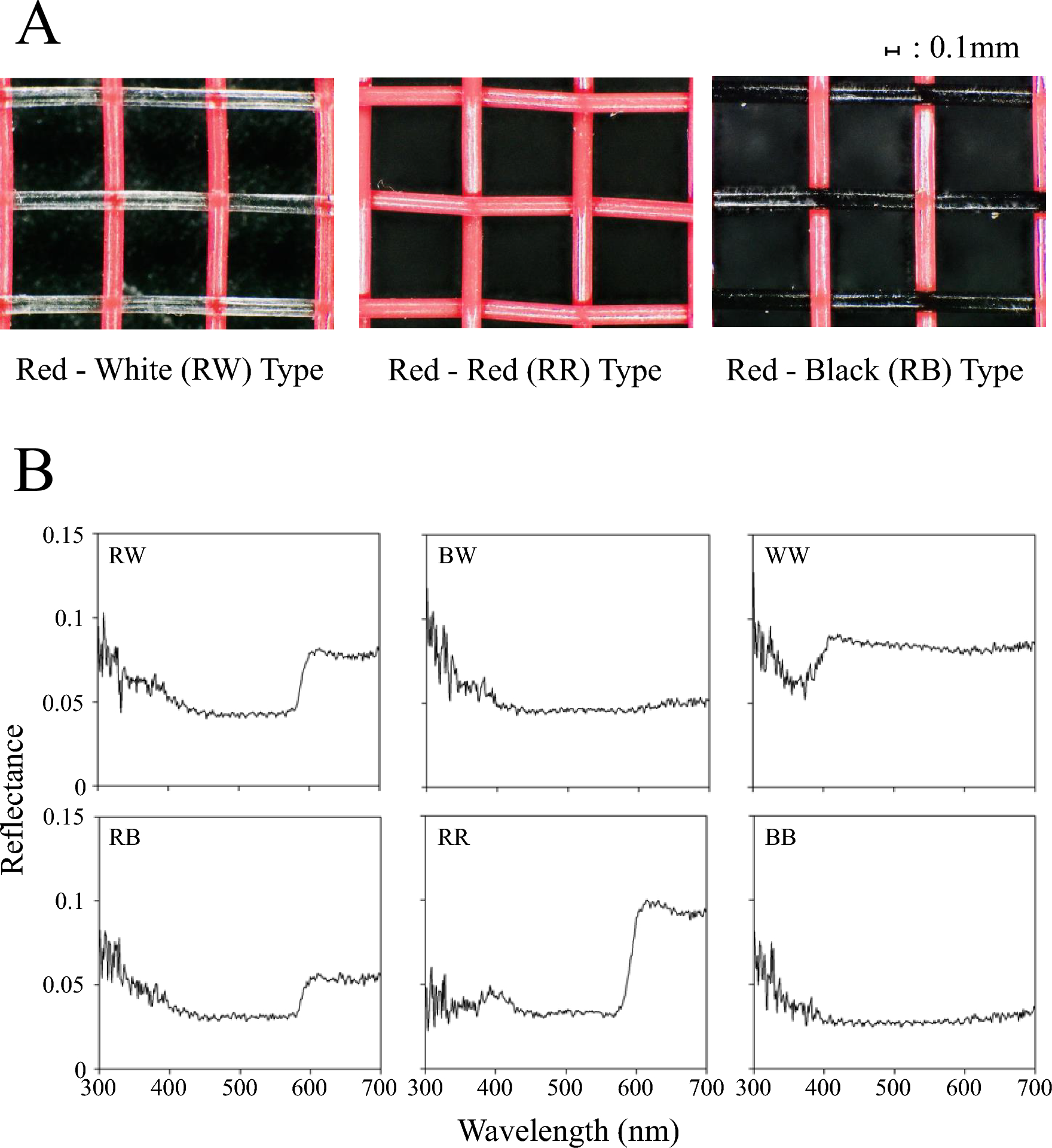The image presents a detailed black and white drawing against a solid white background, displaying two distinct sections labeled "Box A" and "Box B." 

**Box A** features three distinct illustrations of patterns inside rectangular shapes, arranged horizontally. Each pattern corresponds to a different combination and orientation of stripes:
1. The left box, labeled "RW type," showcases red vertical stripes intersecting with white horizontal stripes. 
2. The middle box, identified as "RR type," depicts a dense grid of red stripes crisscrossing in both vertical and horizontal directions, with black filling the intersecting areas. 
3. The right box, marked "RB type," combines vertical red stripes with horizontal black and white stripes.

**Box B** extends below with a more analytical focus, consisting of a 3x2 arrangement of boxes. Each box in this section visualizes the reflectance data through line graphs. The y-axis of these graphs, indicating reflectance, ranges from 0 to 0.15, and the x-axis, denoting wavelength in nanometers, spans from 300 to 700. These graphs are categorized as follows: RW, BW, WW, RB, RR, and BB.

At the top of the image, a scale labeled "0.1 millimeter" is presented, establishing a reference for the depicted patterns. The combination of these visuals delivers an insightful comparative study on the reflectance properties of different striped patterns.